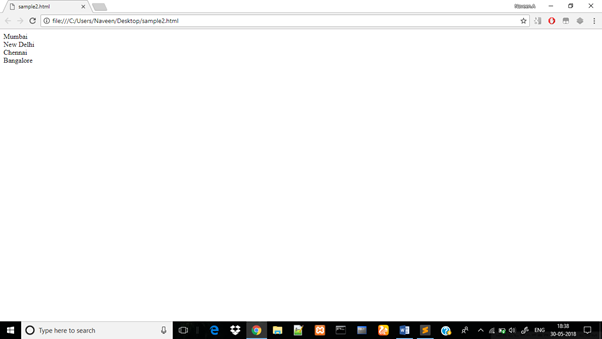Image Description:

The image is a screenshot of a web browser window displaying a website. At the top of the browser, an open tab is visible, featuring an icon of a page with a bent corner and the text "sample 2.html." To the right of the tab's title is a small 'X' symbol used to close the tab.

Below the tab, the browser's navigation bar contains several elements. On the far left are left and right arrows, which are currently greyed out and inactive. Next to these, there's a dark grey refresh button. The address bar itself is white with black text, along with an icon resembling a star on the far right, likely used for bookmarking. Outside the address bar to the right, there are several small icons indicating different browser features.

The main content of the website is displayed below the navigation bar. The website features a clean, white background with black text listing several Indian cities in the following order: "Mumbai" (spelled out as "M-B-A-I"), "New Delhi" ("N-E-W space D-E-L-H-I"), "Chennai" ("C-H-E-N-N-A-I"), and "Bangalore" ("B-A-N-G-A-L-O-R-E").

At the very bottom of the screen, a banner is present, featuring a white square with what appears to be the Windows emblem. To the right of this square is a search bar containing the prompt "type here to search" and a microphone icon representing a voice search option. Below this, there is a black banner displaying various icons, including those for Internet Explorer, an open box, Google Chrome, a folder, and several other small squares with different designs.